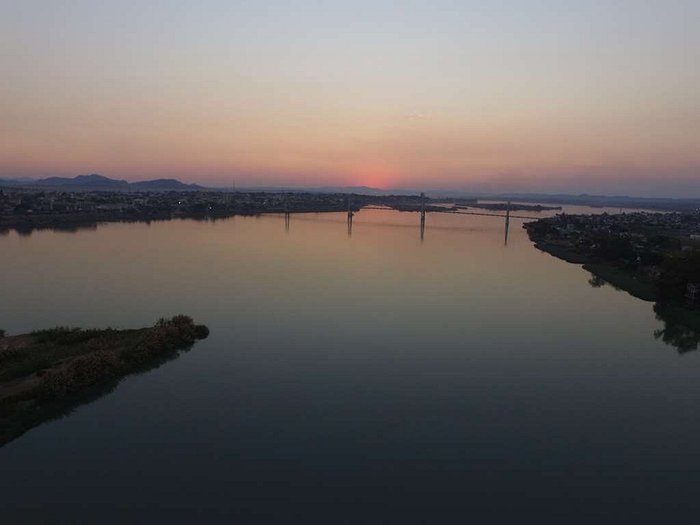A serene and grainy square-cropped photograph captures a tranquil sunset over a murky body of water, possibly a river or lake. The sun, cloaked in a reddish hue, hovers near the horizon amidst hazy clouds, casting a soft light that reflects off the water. Land borders the scene on two sides, forming small peninsulas on the left and right. A bridge stretches across the water in the distance, creating a peaceful silhouette against the sky. Faint, small mountains or hilly terrain add depth to the distant background, contributing to the overall serene and untouched nature of the landscape. The absence of buildings and the presence of fence posts stretching across the water enhance the sense of stillness in this picturesque scene.